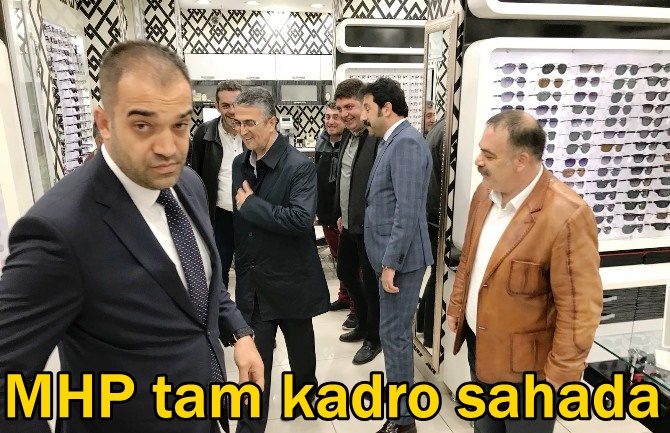The photograph captures six men in a fashionable sunglasses store with a distinct black-and-white geometric patterned wallpaper. On the right-hand side, a balding man with brown hair and a mustache stands in front of a white display case filled with shades of eyeglasses in black, gray, and brown. He is dressed in a tan jacket over a white shirt and dark pants. In the center of the image, a man sporting a blue plaid suit and a mustache stands next to another individual in a black jacket and green top. Beside them, another man in a black jacket and glasses is positioned slightly behind a man wearing a black jacket and a white shirt. On the left side of the image, standing apart from the display, a dark-haired man in a dark suit with a white shirt and a dotted tie looks directly at the camera. Positioned prominently at the bottom of the photograph is a yellow text outlined in black that reads "MHP TAM KADRO SAHADA.” The men, adorned in an array of formal attire, appear to be admiring the sophisticated collection of sunglasses.